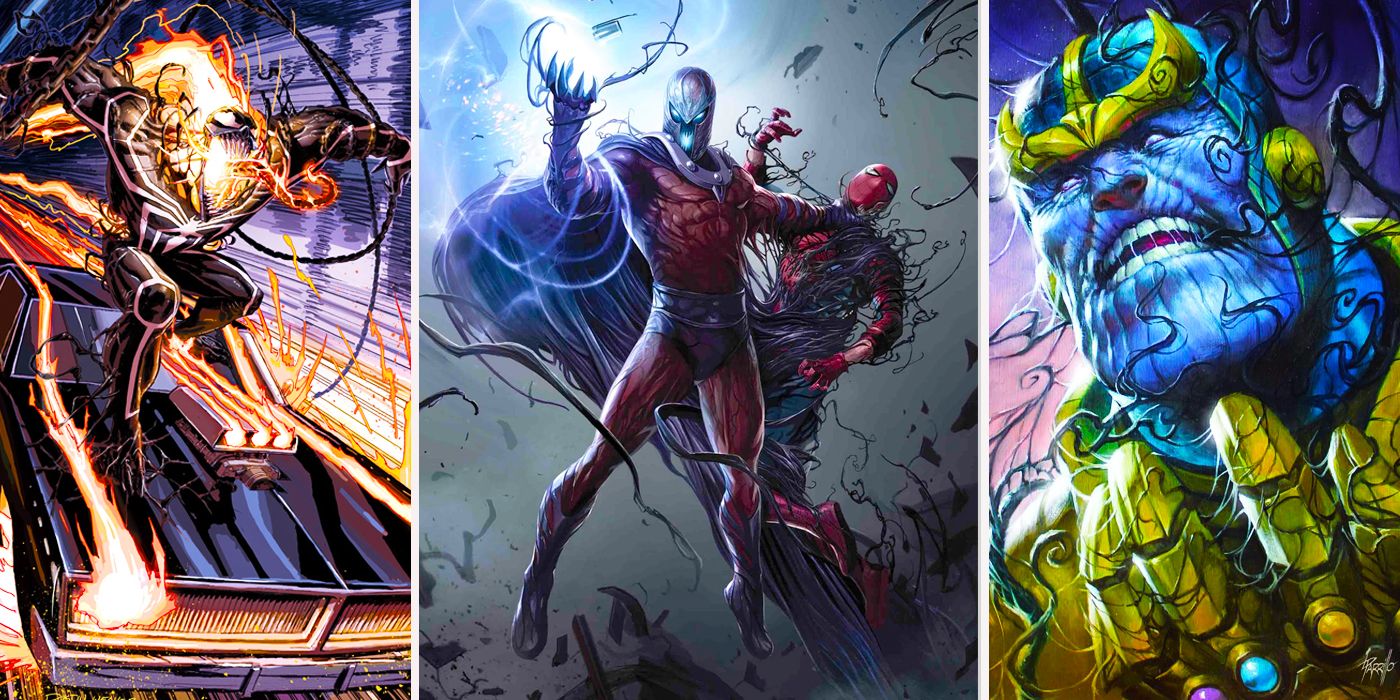The image consists of three comic book character drawings aligned side by side, each occupying an equal third of the image and separated by a small white line. The leftmost drawing depicts a man in a black monster suit with a prominent white spider design on his chest. His head is engulfed in flames, and he has an impossibly large mouth filled with extremely long, finger-length teeth, with a long pink tongue protruding. He is seen riding a black sports car as if it were a skateboard, moving at a high speed with flames and streaks of lightning over the vehicle.

The middle drawing showcases a man in a striking red suit with gray accents, including a belt, boots, and areas around his neck and head. He wears a dramatic purple cape flowing behind him. His right hand is extended forward, emanating light or energy, while his left arm reaches out to grip the neck of another man dressed in a red suit with a face mask, white eyes, and black details around them. This secondary figure appears to be levitating or in mid-air.

The rightmost drawing features a blue-skinned figure gazing slightly to the left. His chin has horizontal lines, and he wears a crown-like adornment with a green emblem on his forehead. Additionally, he has a gold-colored gauntlet on his left hand, prominently displaying three jeweled stones—orange, blue, and purple—on the knuckles. The background of this panel is a blend of light purples and blues with dark, vine-like streaks, adding a dramatic aura. The character's iconic appearance, including the facial features and gauntlet, strongly suggests he is Thanos.